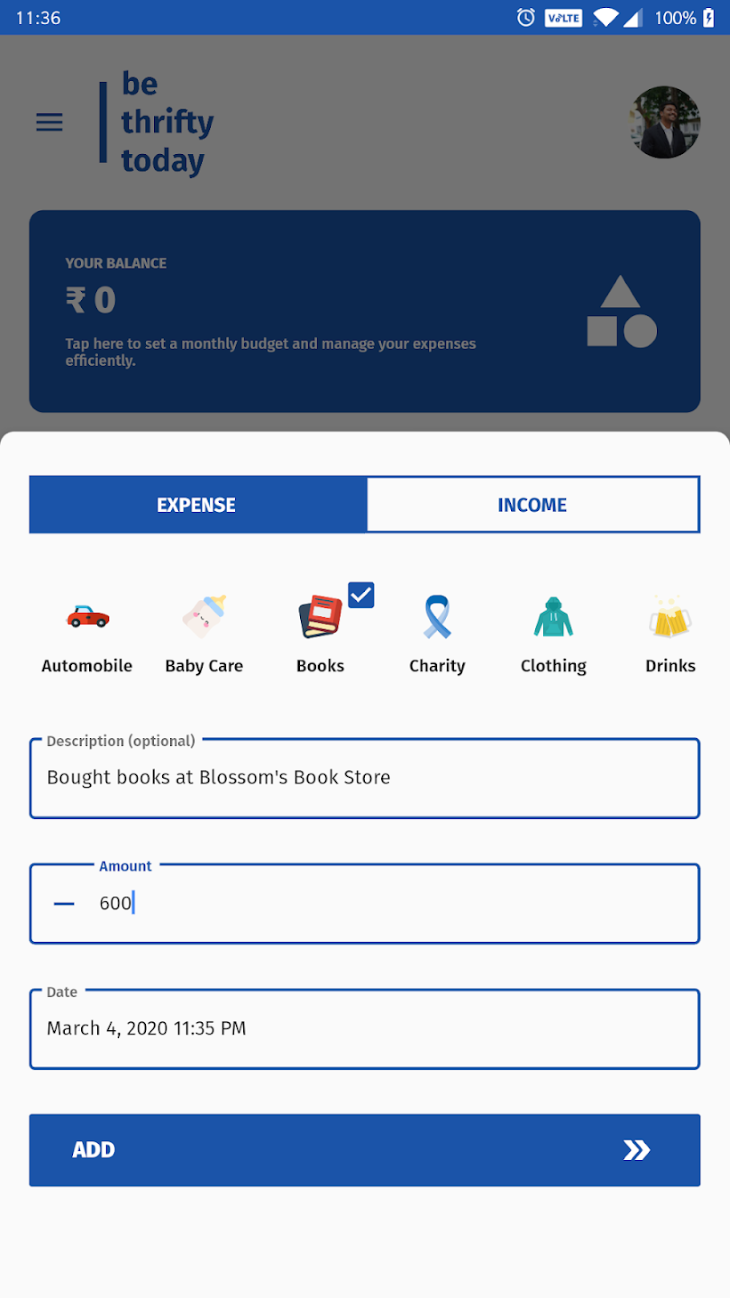This is a screenshot from a cell phone, featuring various interface elements and details across the screen. The top border is about half an inch of dark blue. On the left side, the status reads "11:36," while the right side displays a battery icon at 100% full, three out of four bars for cellular signal, full Wi-Fi signal, a rectangle with "Volt" inside of it, and an alarm clock icon.

Moving to the next section, the screen has a grayish hue, suggesting an overlay or pop-up tab. On the left, there are three horizontal blue lines, each about a quarter of an inch. Next to these lines is a vertical blue line about an inch long. To the right of this, there is text in bold reading "B thrifty today," arranged vertically.

On the left side, there is a profile picture of a man outdoors wearing a black coat and with black hair. 

At the bottom, a blue rectangle spans across the screen with text in white. On the left, it reads "Your balance: $0." Below, in smaller white text, it states, "Tap here to set a monthly budget and manage your expenses efficiently." On the right, there is a segmented icon composed of a white square, a white circle to its right, and a white triangle overlapping both.

Below this segment, the background turns white, with a blue tab on the left labeled "Expense" in white text. On the right, there is a white tab with a blue border labeled "Income" in blue text.

Further down are six icons with matching labels below them: "Auto Meal Bill," "Baby Care," "Books," "Charity," "Clothing," and "Drinks."

Beneath these icons, there is a white rectangle with a blue border labeled "Description (Optional)." Inside, it says, "Bought books at Blossoms bookstore." Below this, another similar bar reads "-600" (indicating an expense amount). Further down, another blue-bordered white tab labeled "Date" contains the text "March 4th, 2020, 11:35 p.m."

At the very bottom, a long blue tab stretches across the screen with the word "Add" in white text on the left, and two thick greater-than signs (>>) pointing to the right.